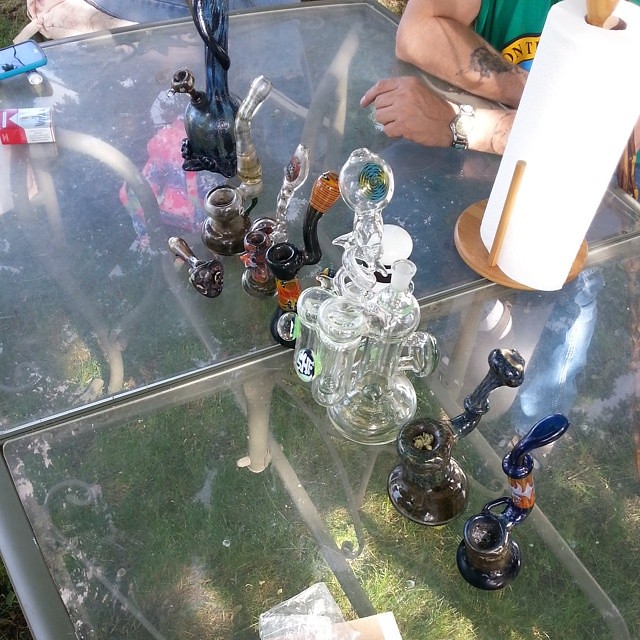In this detailed digital photograph, likely taken inside a store, a glass table that resembles a dining room table dominates the center. The table is supported by either white or silver iron legs and serves as a display for an assortment of marijuana bongs and pipes, meticulously arranged vertically. Starting from the left, one of the bongs is blue with a dark greyish bottom and blue handle. Beside this, there is another with a greyish top and bottom. A series of clear glass pipes follow in the middle, flanked by a light brown one with a dark grey hook. Next to them, a silver bong and another darkish grey one complete the lineup.

To the upper left of the table, a pack of Marlboro cigarettes with its distinctive red and white packaging is noticeable. On the right side, a Caucasian man wearing a sleeveless green t-shirt with a tattoo on his left arm and a wristwatch on his right sits at the table. His shirt features a yellow spot with black lettering. Adjacent to him is a white paper towel roll mounted on a brown dowel paper towel holder. The overall scene is enriched by the detailed display of smoking paraphernalia and hints of the store’s ambiance, framed by the casual presence of the man to the right.